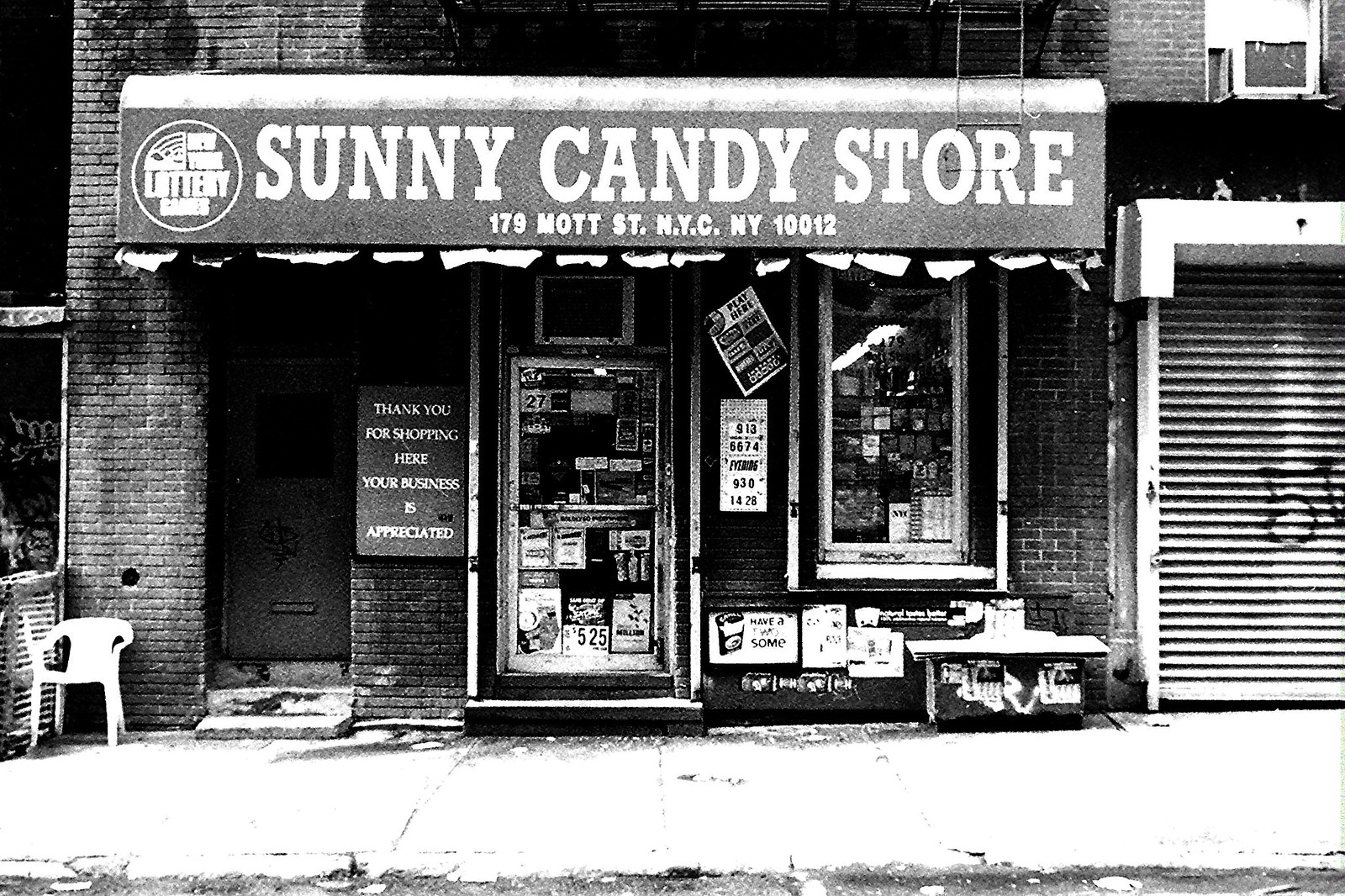This black-and-white outdoor photograph captures the storefront of the Sunny Candy Store, located at 179 Mott Street, New York City, NY 10012. The brick building features a banner at the top that clearly reads "Sunny Candy Store," with smaller text beneath it displaying the address. To the left, a white plastic chair sits at the entrance, subtly inviting passersby. The storefront window and door are cluttered with a variety of stickers and posters, one of which includes an advertisement for Camel cigarettes. Prominently displayed next to the door is a sign that reads, "Thank you for shopping here. Your business is appreciated." On the far right side of the image, a corrugated metal roll-down door is visible, spray-painted with the number '5'. The store fronts onto a pavement that extends to the right towards another storefront with its metal closure down.